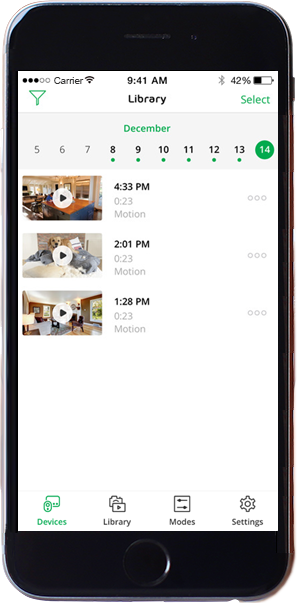The image displays a digital interface, likely from a smartphone or tablet, framed by a black border on all sides. In the top-left corner, there are three black circles, followed by two white circles. To the right of these, the word "Carrier" is prominently displayed. Next to this, a WiFi signal icon can be seen. Centered at the top of the screen is the current time, "9:41 AM." Below the time, the word "Library" is written. On the far left, there is a green icon resembling a clothes hanger, while the top-right corner features a Bluetooth symbol and a battery indicator reading "42.9%." Beneath the battery percentage, the word "Select" is displayed in green.

Below this header section, a light gray area features "December" written in green at the center. This segment outlines the calendar days from 5 to 14, with small green circles under each day from 8 to 13. The 14th day is highlighted with a large green circle encircling the number 14.

Underneath the calendar section, there are three video thumbnails aligned horizontally, with corresponding timestamps displayed on the right side of each thumbnail.